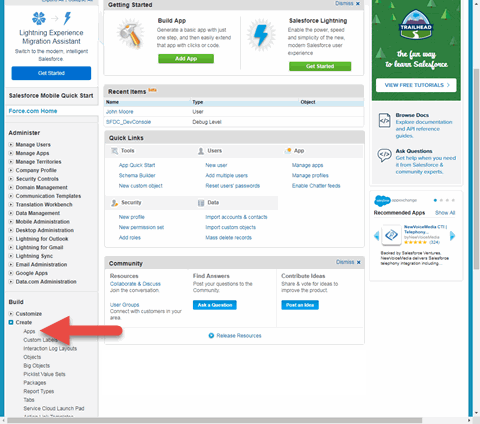Screenshot of a Salesforce Interface with Expanded 'Create' Section in 'Administer' Menu

The image is a screenshot of a Salesforce interface, which is visually divided into three main sections. 

On the left is a navigation menu that lists various modules and tools available to the user. At the top of this menu, "Lightning Experience Migration Assistant" is prominently displayed, likely as a high-priority task or tool. Beneath this, there are menu items like "Salesforce Mobile Quickstart" and "Force.com Home," followed by an "Administer" section containing multiple expandable options such as "Manage Users" and "Manage Apps," among others. This section is extensive and continues with additional subcategories.

Next, in the middle section of the screen, the "Administer" menu reveals more detailed options after expanding. Specifically, the "Create" section is opened, displaying a list of sub-options including the creation of apps. At the top of this sub-section, there is a "Getting Started" guide, followed by links to recent items, quick links, and community resources.

The organization and labeling of these sections highlight the structured and hierarchical nature of the Salesforce interface, designed to guide users efficiently through various administrative and development tasks.